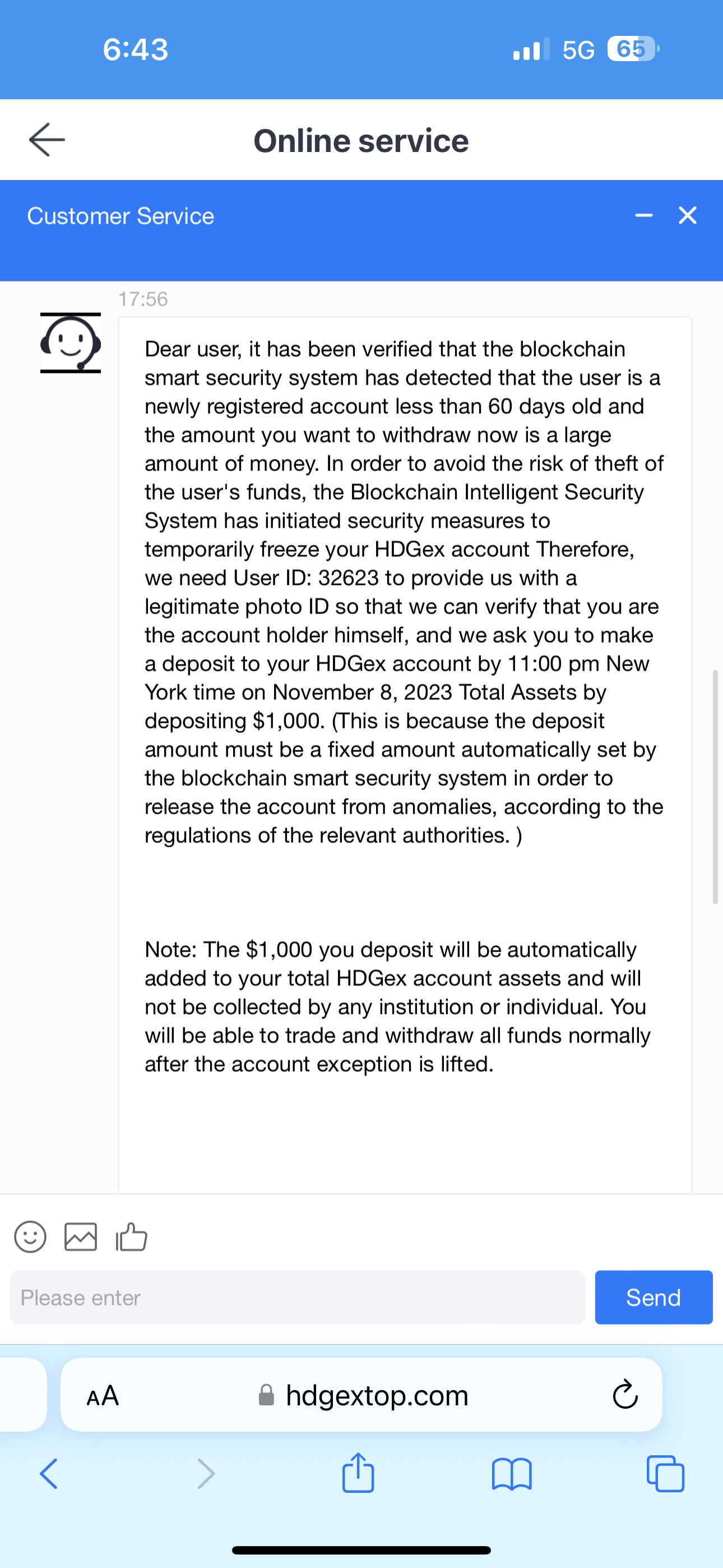**Caption:**

The image on the phone screen displays a message from an online service's customer support. The message indicates that the user's account has been verified through a blockchain smart security system. However, because the account was newly registered with a high amount of $60,000 for withdrawal, security measures have been triggered. The system has temporarily frozen the user's account and requires additional verification.

The customer support message explains that to proceed, the user must provide proof of identity. Additionally, they must make a fixed deposit of $1,000 to confirm their legitimate ownership of the account. This deposit will be added to the user's total assets and will not be available for immediate trading or withdrawal until verified.

In essence, the message informs the user that their large withdrawal request has been flagged due to the newness of their account and the significant amount involved. The security protocol mandates a deposit and identity verification to prevent potential fraudulent activity. The overall tone suggests caution and adherence to regulatory standards, though the user expresses confusion and frustration over the additional requirements for accessing their funds.